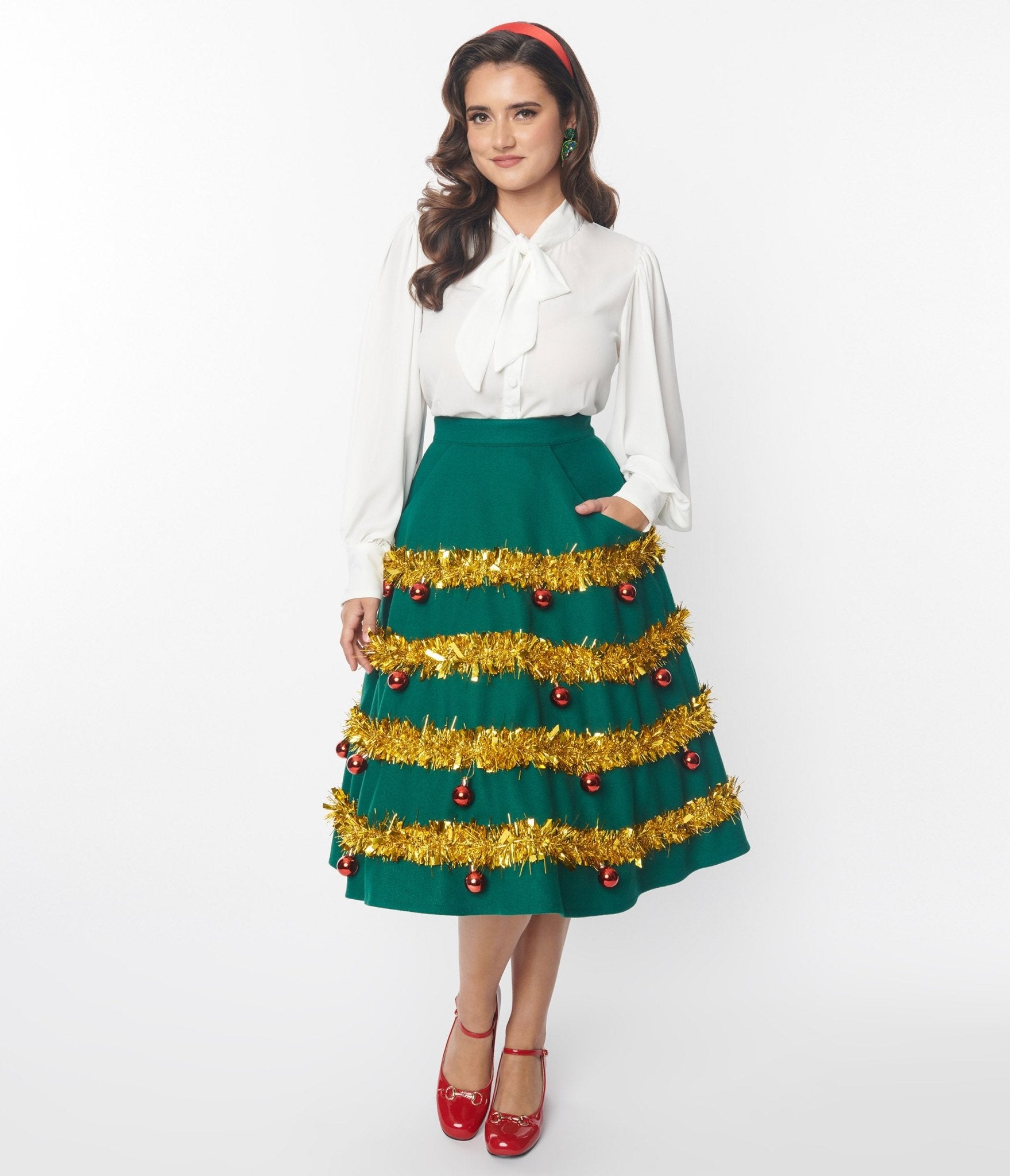In the image, a young woman stands against a gradient background that transitions from white at the top to a darker gray at the bottom. She has long, wavy dark brown hair adorned with a red headband, and wears green jade earrings, with only the left one visible. Her thick eyebrows and dark eyes are complemented by a wide smile, a large forehead, and a widow's peak with her hair parted at the crown.

She is dressed in a white long-sleeve blouse, which features a loosely tied scarf at the neckline. Her left hand is casually placed in the pocket of her green skirt, while her right arm rests by her side. The green skirt, designed to resemble a Christmas tree, is embellished with four rows of gold tinsel, from which hang red ornaments.

Completing her festive look, she wears red patent leather strappy high heels that fasten around her ankles. The overall ensemble gives a celebratory and seasonal appearance, enhanced by the decorative elements of her outfit.